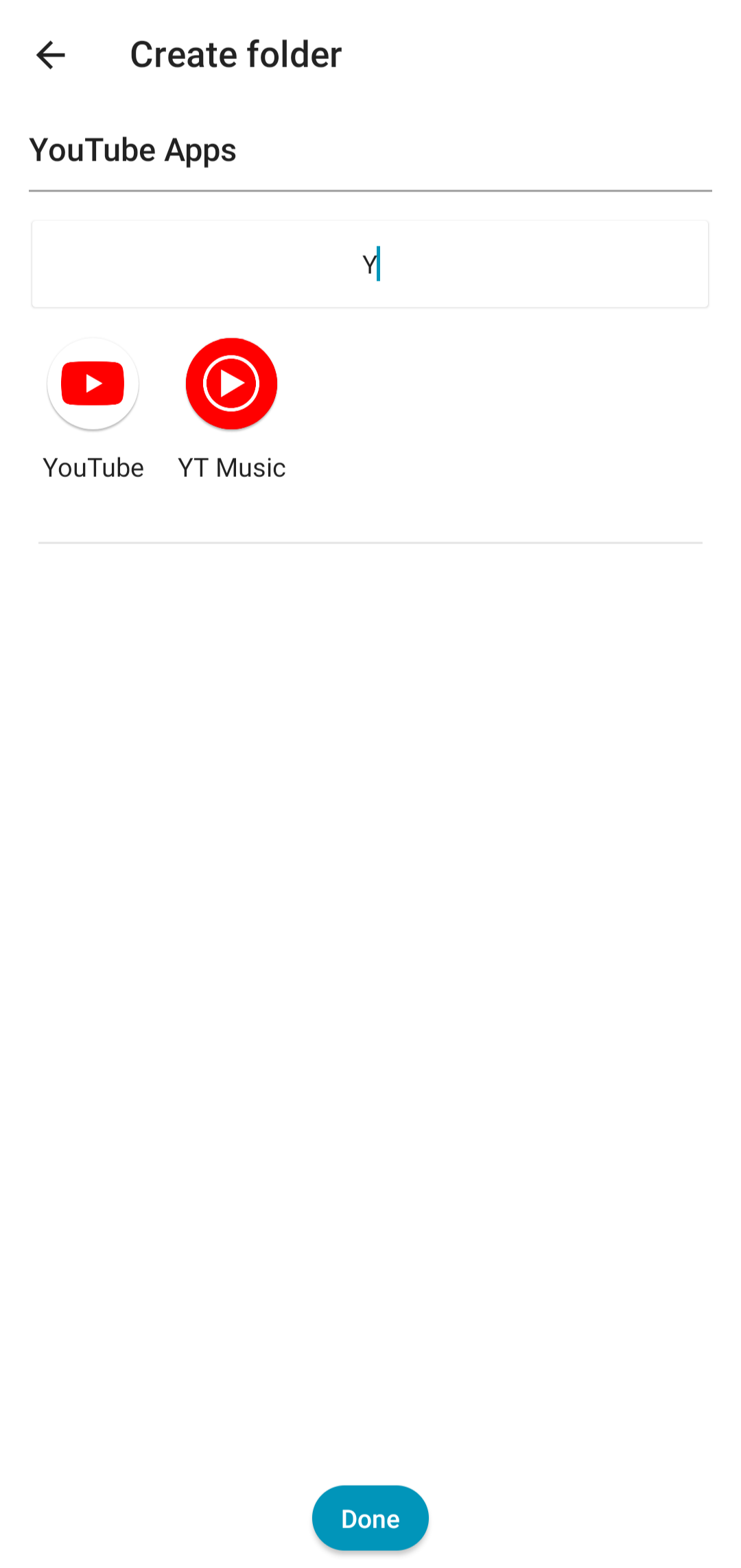The image captures a minimalist screen within a smartphone's settings interface, predominantly white, focused on the task of creating a folder specifically for YouTube-related apps. At the top of the screen, a black back arrow points left, indicating the option to return to the previous settings menu. Adjacent to this arrow are the words "Create a Folder."

Occupying the central part of the screen is a small, capital "Y" in a light font, accompanied by a short vertical blue line signifying the text cursor, suggesting the space is ready for input. Below this text entry field, on the left side, is the familiar YouTube icon—a red rectangle with a white play button centered inside it. This icon is slightly circled, set against a small white button backdrop, labeled "YouTube."

Next to it, in a similar fashion, is another circular icon, this time in solid orange with a white play button, identified as "YT Music." At the very bottom of the screen, a "Done" button is present, indicating the action to finalize the creation of the folder.